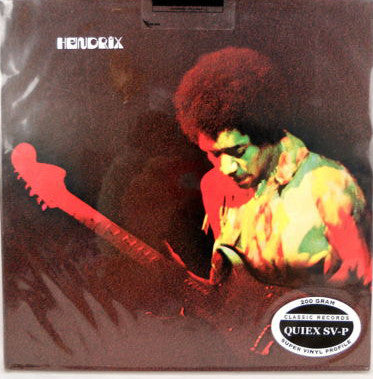This is the front cover of the iconic Jimi Hendrix album "Band of Gypsies." The cover features a partially profile view of Jimi Hendrix, dressed in a vibrant tie-dye shirt with red, yellow, and green tones, and his signature afro hairstyle. Hendrix is captured in an intense moment as he plays his guitar, his hand poised on the frets. The background of the image is a deep black, emphasizing the vivid colors of his shirt and the red hue of his guitar neck, cast by stage lights. The top left corner of the cover is adorned with the word "Hendrix" in large, stylized white letters. The bottom right corner features a black and white sticker that reads "300 Grain Classic Records, Quiex SVP." The album cover itself is seemingly preserved under a clear plastic wrap, highlighting its status as a coveted collector's item.